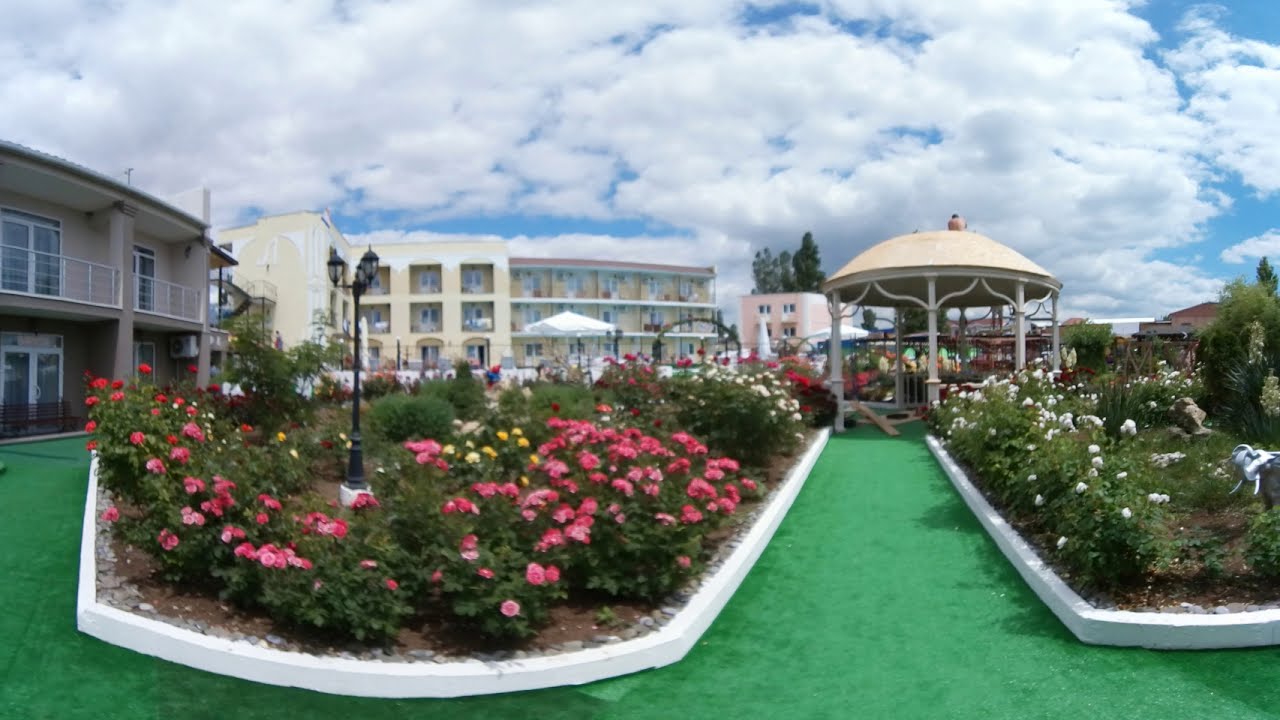The image depicts an outdoor walkway carpeted with a bright green turf that extends into the distance, curving to the right and also branching out to the left, framed by white-trimmed edges. Flanked by large garden beds encased in small white barriers, the left garden showcases vibrant pink, yellow, and red flowers, accompanied by a small black lamppost, while the right garden is adorned with white flowers and abundant greenery. At the far end of the walkway sits a white, ornate gazebo or awning with a rounded dome top. In the background, multi-story buildings are visible: a prominent yellow three-story building, possibly an apartment or hotel with equally spaced windows, doors, and small balconies, and further left, the corner of a two-story brown building. Above, the bright blue sky is partially obscured by large, fluffy white clouds, creating a picturesque backdrop.